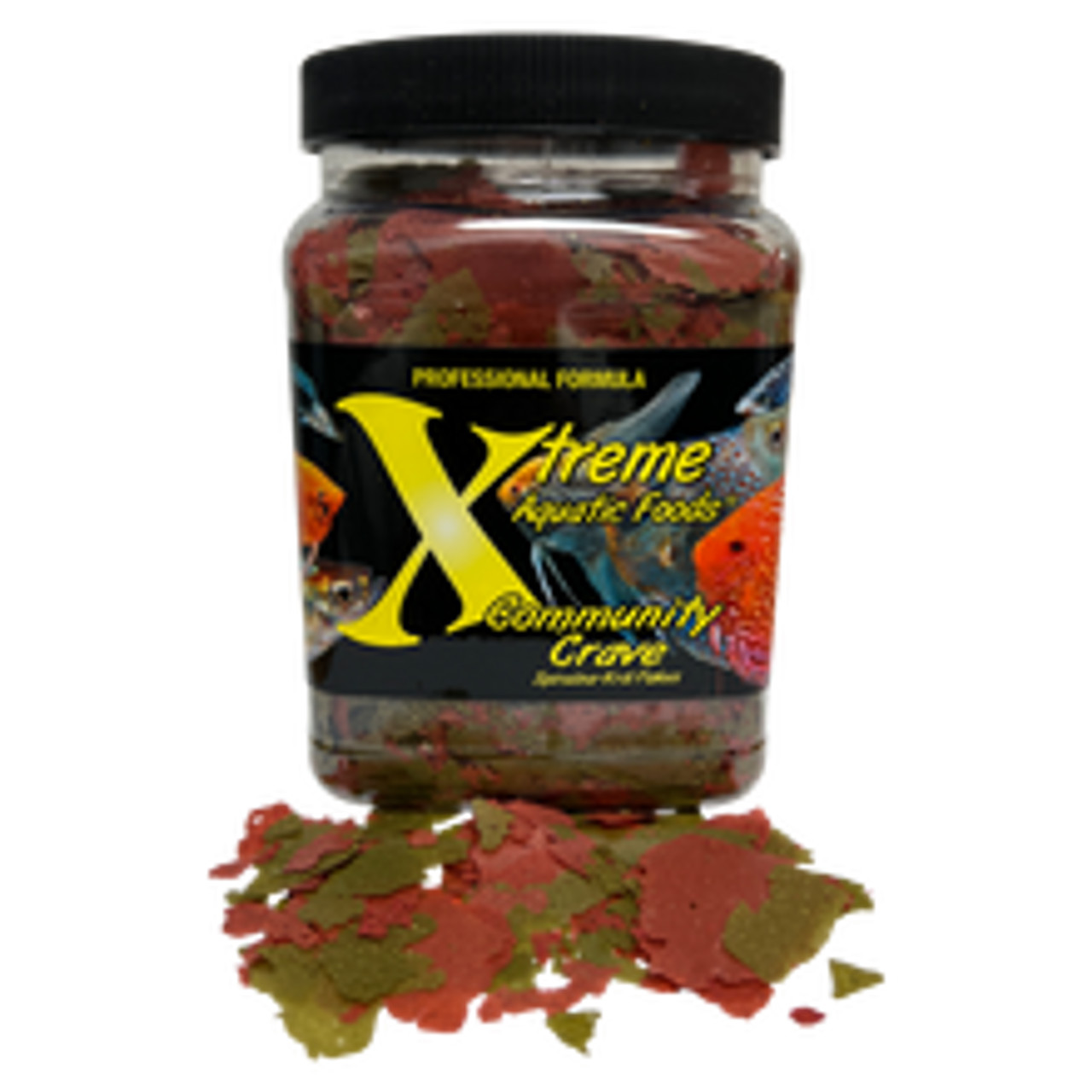The image features a clear plastic jar with a black lid and a prominent black label across the center, set against a plain white backdrop. The label displays "Professional Formula" and "Extreme Aquatic Foods, Community Crave" in bright yellow font. Illustrations of colorful fish, resembling bettas in hues of orange, blue, and possibly turquoise with stripes, swim across the label. The jar contains a mix of dark red and green fish food flakes, some of which have spilled onto the surface below. The flakes inside and outside the jar are varied in size, ranging from large pieces to smaller, broken bits. The overall appearance evokes the look of autumn leaves due to the rich, earthy colors of the flakes.